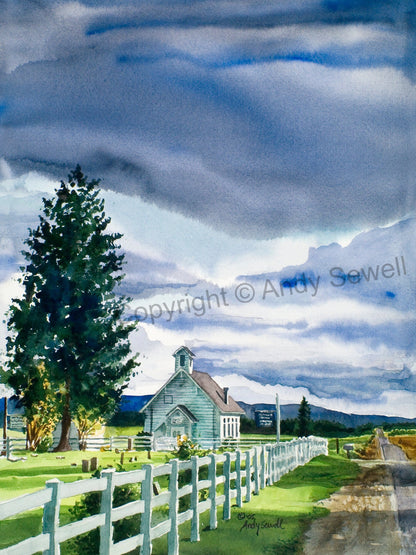The watercolor painting by Andy Sewell depicts a serene country scene dominated by a light blue sky with thick gray clouds and hints of blue peeking through. In the center of the image stands an old, small, white church with a red roof, featuring a bell tower and a dormer roof above its doors. Four windows line one side of the church. Surrounding the church is a white picket fence, which encloses a yard that contains green bushes and what appears to be a small graveyard with tiny tombstones and markers. On the right-hand side within this yard stands a very tall fir tree, at least twice the height of the church, with an illegible sign nearby.

In front of the church and extending toward the horizon runs a country road, bordered by a grassy area that transitions from dirt to lush grass. Adjacent to the road and inside the yard is a mailbox for the church, and further down the road, there's another building and a white sign with blue lettering. Mountains can be seen faintly in the distant background, enhancing the picturesque countryside setting. The composition is nostalgic, reminiscent of scenes from a storybook, capturing the tranquil essence of rural life.